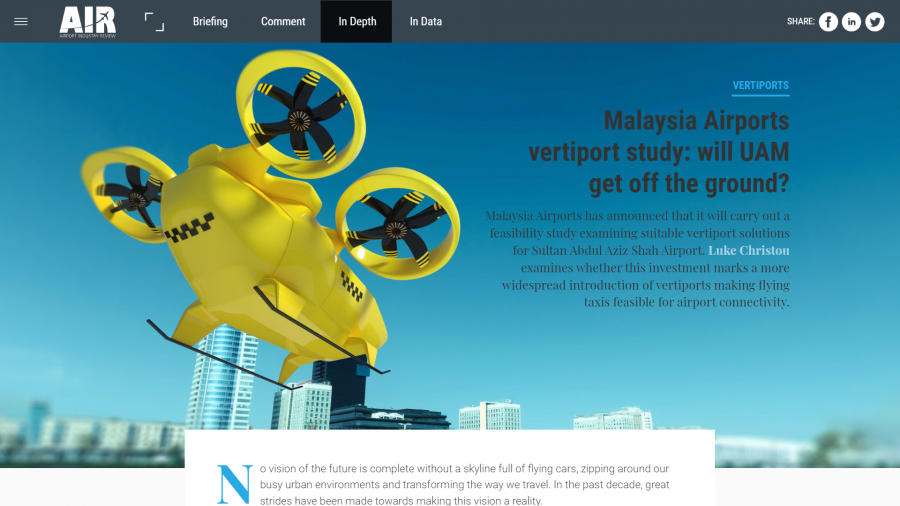**Descriptive Caption:**

This image is a screenshot of the Air website, showcasing its clean and organized interface. The top portion of the screenshot features a navigation menu that doubles as the website's header. On the upper left-hand side, a hamburger menu icon is situated next to the company's logo— the word "Air" in bold white font with a miniature airplane flying across it, emphasizing the site's aviation focus.

The navigation menu includes several links: "Briefing," "Comment," "In-Depth," and "In-Data," catering to various content sections. On the far right side of the menu, there are buttons for sharing content, enhancing user engagement.

Below the navigation menu, the background transitions to an image of a vibrant yellow drone soaring through the sky, set against a sprawling cityscape. To the right of the drone, a featured article is prominently displayed. The headline, "Malaysia Airport Severity Port Study. Will UAM get off the ground?" is written in bold black text, intriguing the reader with a critical question on urban air mobility (UAM).

Below this headline, a brief teaser text introduces the article, captivating the audience's curiosity. At the bottom of the image, a white rectangle with additional information is partially superimposed over the cityscape backdrop, offering further context about the featured article. This detailed layout ensures a visually appealing and informative experience for the user.